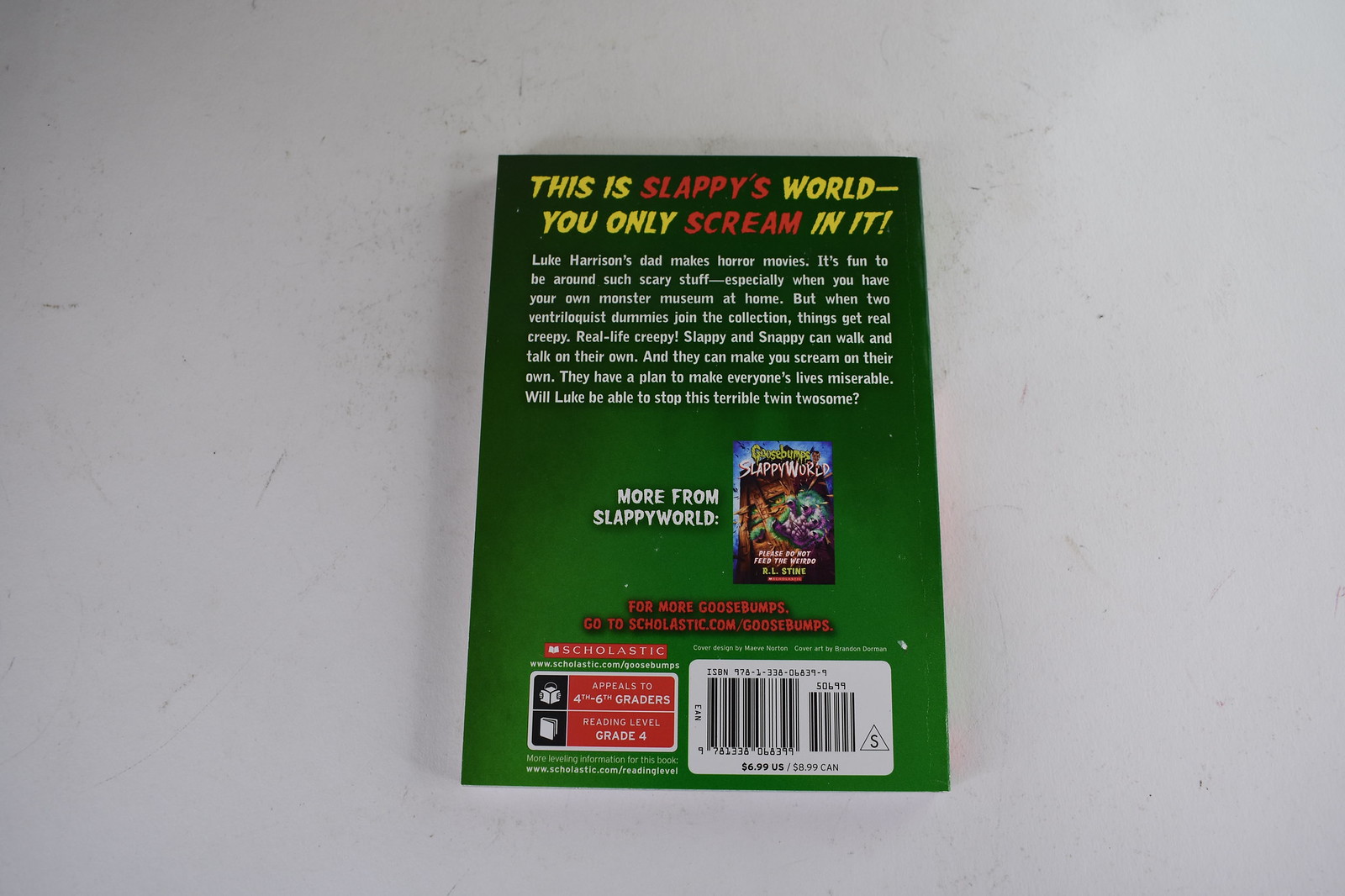The image shows the back cover of a Goosebumps book from the "Slappy's World" series. The background is green, resembling green smoke. The main text, written in a mix of yellow and red fonts, reads "This is Slappy's world. You only scream in it." Below that, the book description provides the following eerie summary: "Luke Harrison's dad makes horror movies, and it's fun being around such scary stuff, especially when you have your own monster museum at home. But when two ventriloquist dummies, Slappy and Snappy, join the collection, things get real creepy. They can walk and talk on their own, and they have a plan to make everyone's lives miserable. Will Luke be able to stop this terrible twin twosome?"

The author's name, R.L. Stine, is printed at the bottom of the cover, and below that, there’s a call to action in red text: "For more Goosebumps, go to Scholastic.com/goosebumps." The bottom left of the cover features the Scholastic logo and a square label indicating the book appeals to fourth to sixth graders, with a reading level marked as fourth grade. To the right, there’s a white and black barcode. The cover also includes a promotional image for another book in the "Slappy's World" series, advertised just below the main description. The book itself appears to be placed on a marble or scuffed floor, indicated by its white background with black scratches.